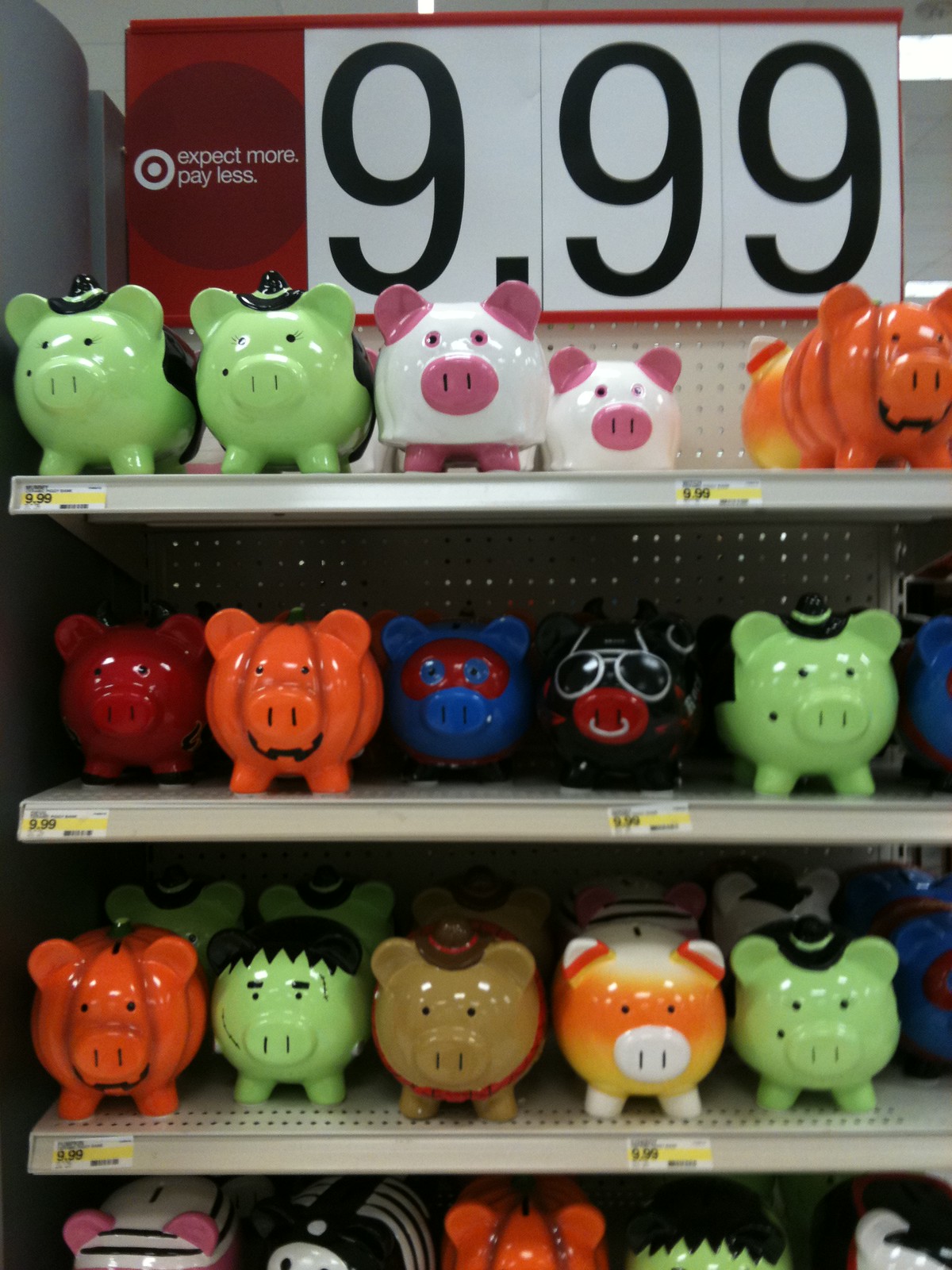This detailed, realistic photograph captures a vertical section of a display at a Target store. The focus is on four light gray shelves, which occupy the bottom three-quarters of the image, each adorned with a variety of decorative piggy banks, all facing forward. The store's light gray ceiling is visible above. At the top of the image, a red banner with a white Target logo and the slogan "Expect More, Pay Less" is prominently displayed. Adjacent to this, large white signs with the price "$9.99" are visible.

Each shelf showcases an assortment of Halloween-themed piggy banks, featuring an array of vibrant colors and playful designs. On the top shelf, green pigs wearing black witch hats are positioned next to pigs designed to resemble ghosts with white sheets. The second shelf includes red pigs with devil horns, pumpkin pigs, a blue Superman pig with a red mask, and more witch-themed pigs. One pig with glasses is partially out of view. The third shelf displays pumpkin pigs, a green Frankenstein pig with jagged black hair, a tan pig with a small hat, and a candy corn pig with orange, yellow, and white stripes. Amidst these are more witches and a jumbled group of variously colored pigs. The bottom shelf, though only partly visible, features a black pig with white skeleton ribs and a partial skull face.

The shelving units are silver on the sides, and a white pegboard with holes forms the backdrop of the display. Vertical white stickers with yellow stripes and illegible prices are affixed to the sides of the shelves. The overall setup suggests a seasonal Halloween display, complete with creatively themed piggy banks ready for purchase.